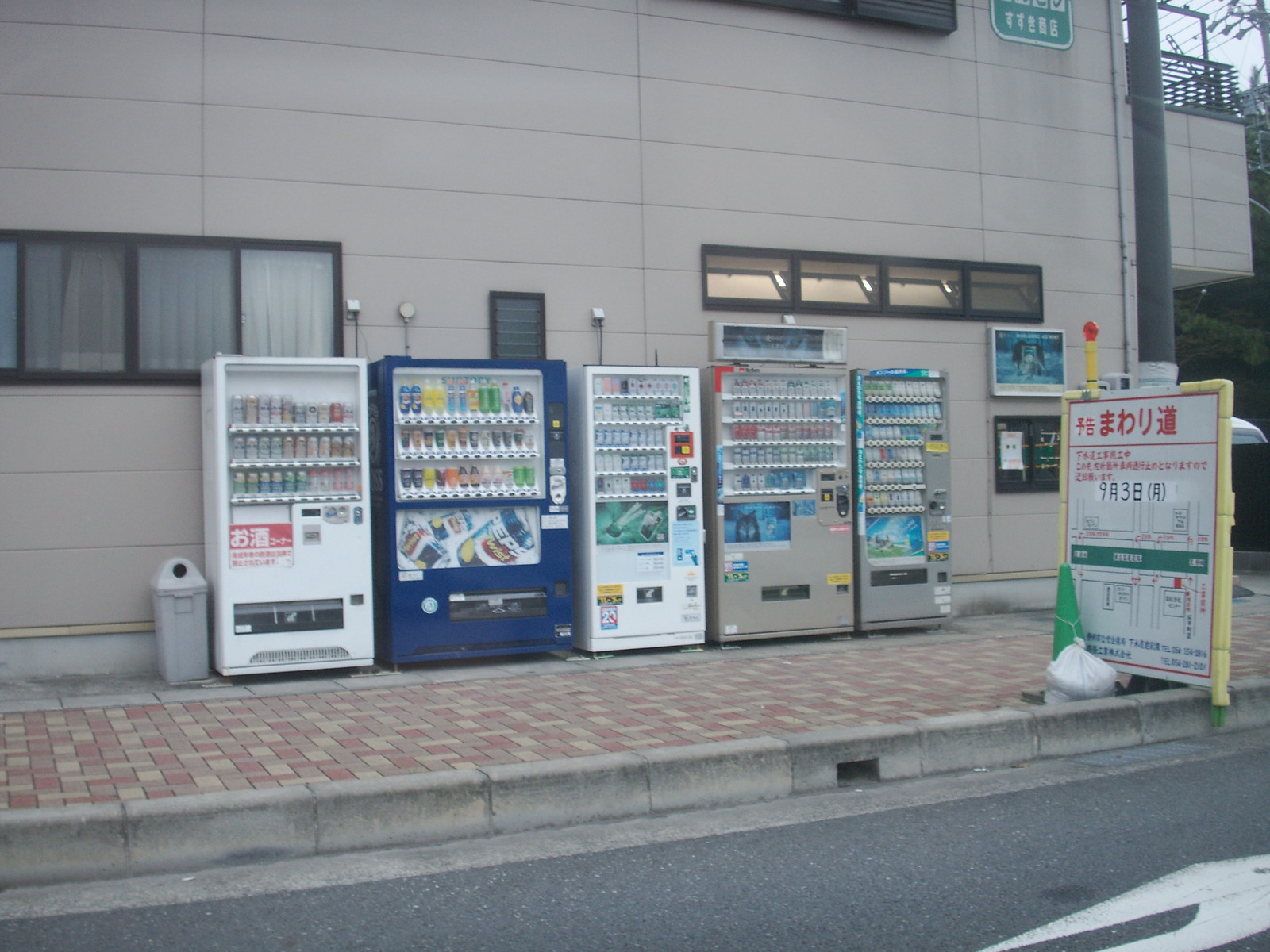The photograph depicts a bustling street scene in an Asian city, likely Japan, featuring five vending machines lined up against a tan, rectangular building with two visible black-framed windows. The building faces a sidewalk made of three different colors of brick, arranged in a geometric pattern, and is bordered by an asphalt road in the foreground. The vending machines, appearing to vend a variety of beverages in bottles and cans, are aligned from left to right: the first and third machines are white, the second is blue with prominent Pepsi signage, and the fourth and fifth have a stainless steel finish. To the left of the vending machines stands a small gray trash can with a circular opening. On the far right side of the image, a light post features a sign with red Chinese characters set against a white background with yellow sides.